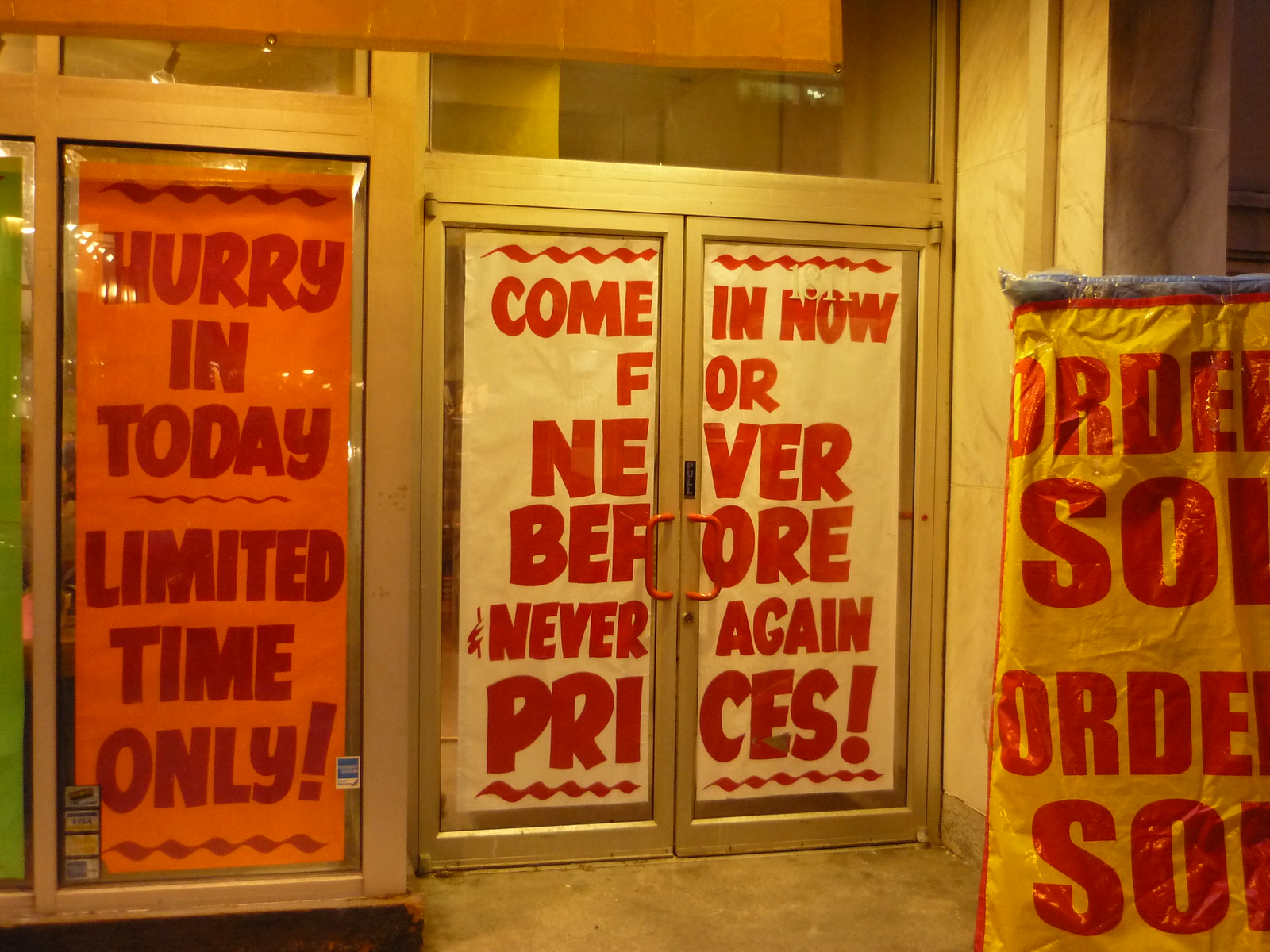This photo captures the storefront of a commercial establishment. Dominating the center is a closed door with a clear glass window, which is almost completely obscured by a prominent yellow sign. The sign reads, "Come in now for never before, never again prices." Flanking the door, the window on the right features an orange sign that urges, "Hurry in today," with the additional message, "Limited time only!" underscored below. To the left of the door, there is a partially obscured sign that appears to instruct customers to "Order soon," though some of the text is blocked from view.